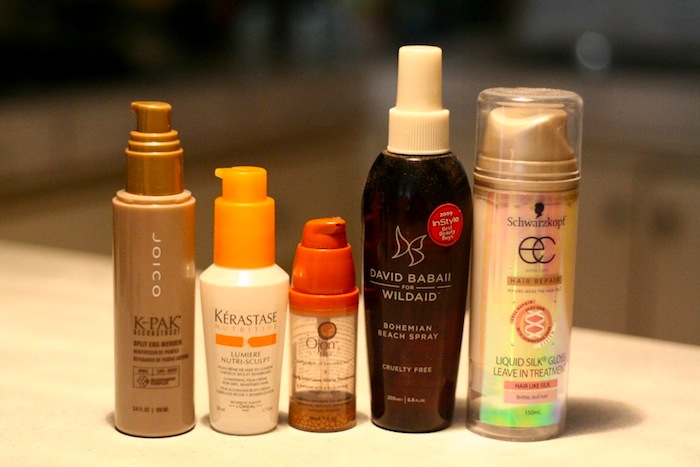This photograph showcases an array of beauty products meticulously arranged in a horizontal line on a beige countertop. The background of the image is blurred, featuring a dark countertop on the left with a light backsplash, transitioning into a shadowy upper section, while the right side subtly reveals part of white cupboards. 

The foreground is dominated by five distinct bottles: 

1. On the far left, there is a tall, light brown plastic bottle with rounded vertical edges. It has a matching brown pump and is adorned with white and black text.
2. Adjacent to it stands a shorter, round, white plastic bottle, equipped with an orange pump. It features black writing, prominently displaying "Kérastase" at the top, followed by two orange rectangles.
3. The third bottle is transparent, revealing an amber liquid inside. It has a red pump, and near the top, there is a brown-outlined circle filled with a red-orange hue.
4. Next, there is a tall, brown bottle that broadens at the top, capped with a white pump. It carries white text and sports a circular red sticker with white writing on the right-hand side.
5. The final bottle on the right is a clear, tall, round container with "Schwarzkopf" inscribed at the top in black. It holds a light yellow cream and is topped with a gold pump, protected by a white plastic cover.

The composition of the photograph, though blurred in the background, brings detailed attention to the varied shapes, colors, and branding of the beauty products in the foreground, meticulously highlighting their distinct characteristics.